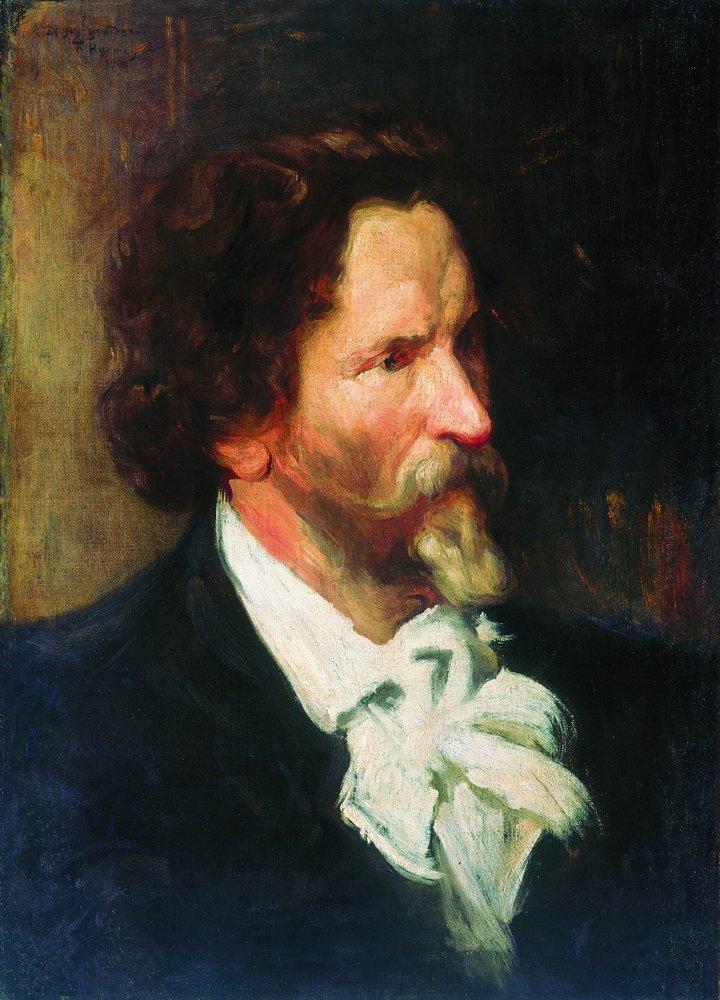The image is a portrait painting of a man from either the 18th or 19th century, capturing a side profile as he looks off to the right. His face, partially turned, reveals a long, prominent nose, and blue eyes. His complexion is light, with a hint of reddish undertones. He has dark brown, slightly curly hair that falls just behind his earlobe. His facial hair includes a thick, white beard and mustache, adding a distinguished touch to his appearance. He wears a white, ruffled shirt with an elegant ascot around his neck, beneath a dark blue jacket or vest. The background is split into varying shades of dark colors: light brown on the left, blending to dark brown or gray in the middle, and turning darker towards the right where two indistinct figures appear to be standing in the background.